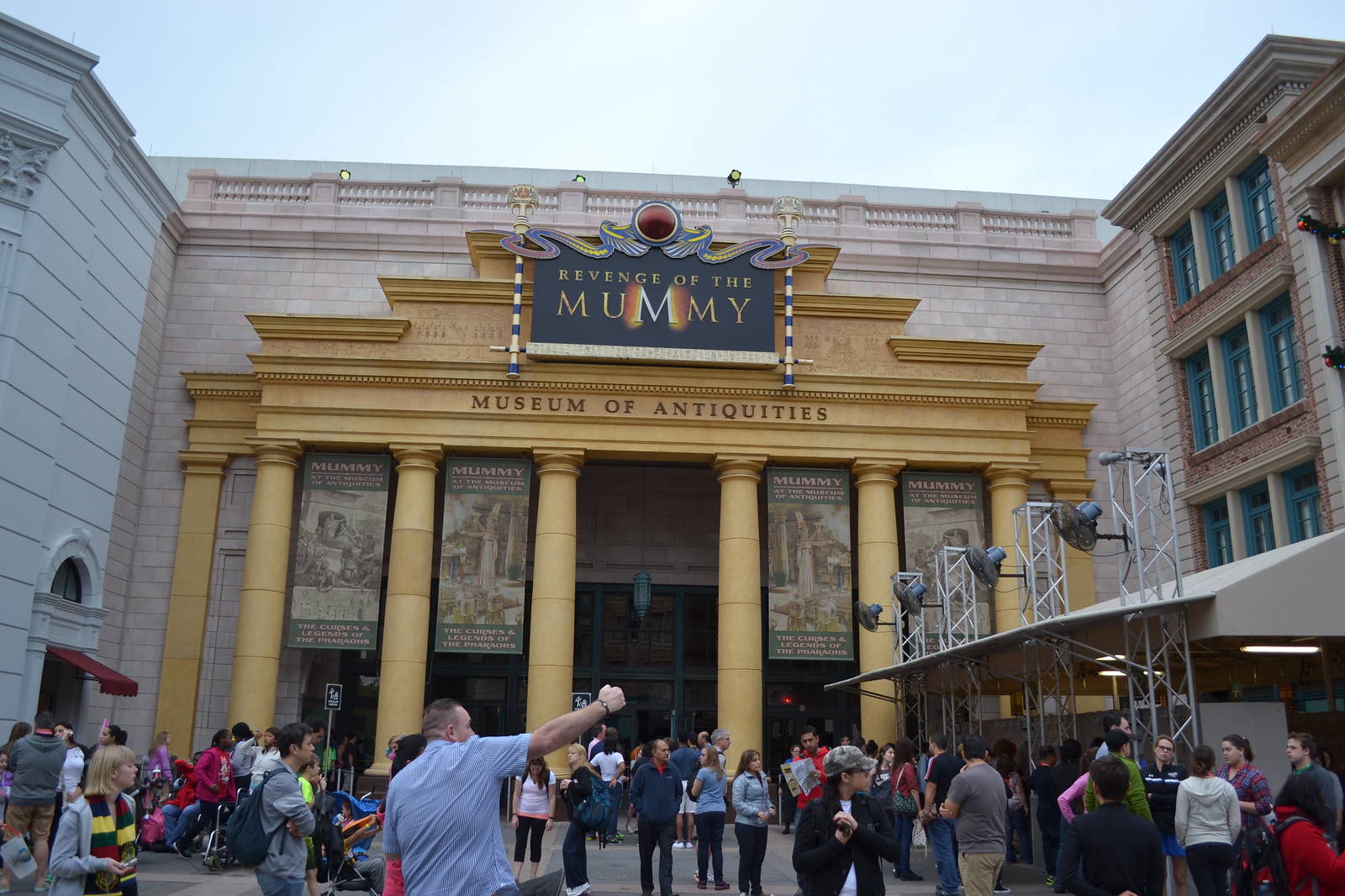The image depicts the front of a museum designed to resemble an ancient Greek structure, albeit with largely fake elements. The museum's facade is painted gold and features four large banners hanging from windows at the top. The central black banner prominently reads "Revenge of the Mummy" in gold lettering, while, below on the building itself, raised black letters spell out "Museum of Antiquities." The entrance is adorned with tan-colored pillars and surrounded by gray stone or brickwork. In the courtyard, multiple people are gathered, many dressed in long sleeves and pants, suggesting a cool, overcast day. To the right, there's a covered tent area with silver scaffolding, housing fans and illuminated by fluorescent bulbs. The front also boasts large glass windows framed in green.